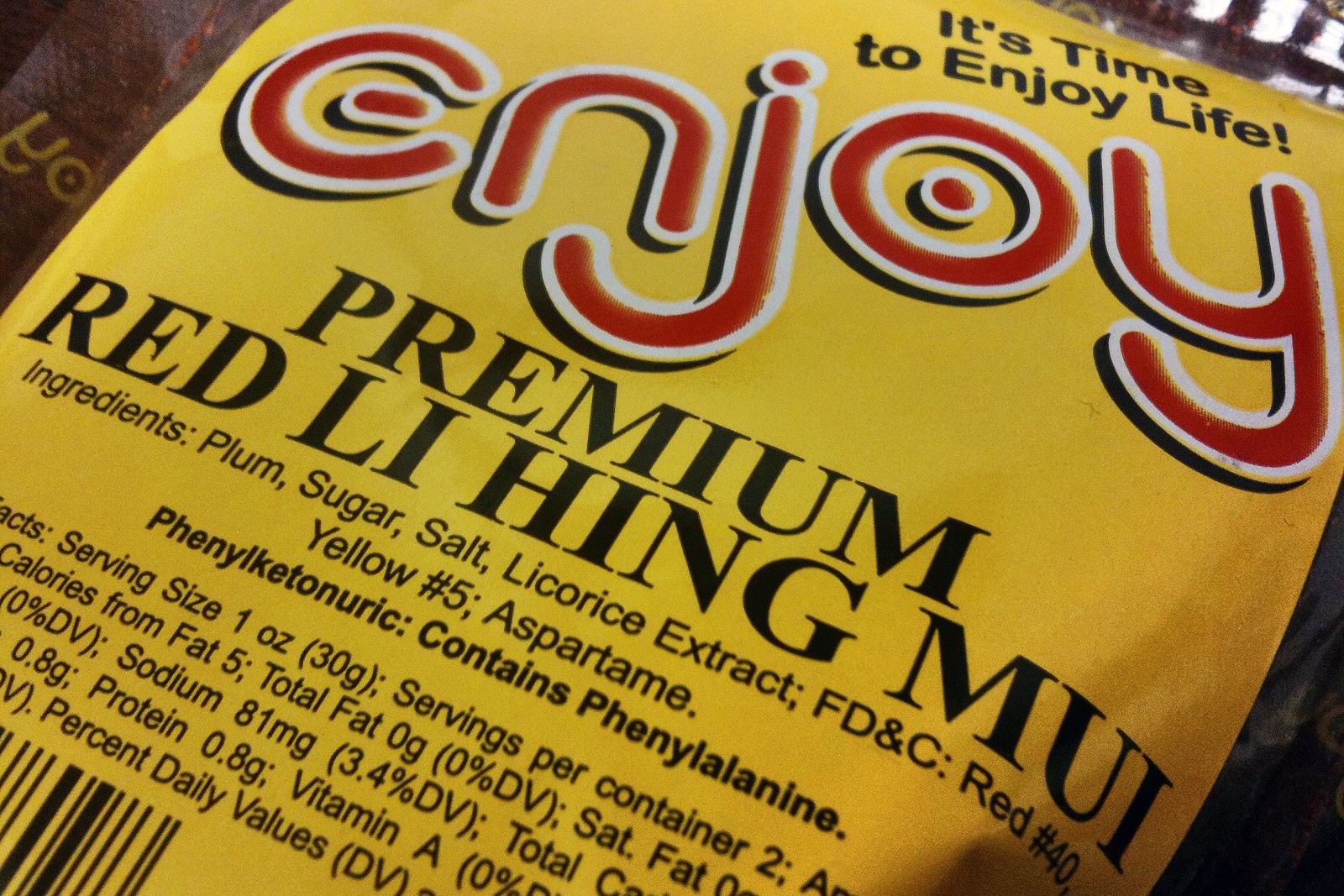The image depicts a yellow food package adorned with black and red writing. Prominently at the top right, it declares in bold black text, "It's time to enjoy life." Just below this, stretching across the top in large, white-outlined red letters, is the word "Enjoy," with a small dot inside the "O." Centrally placed in the image, "Premium Red Li Hing Mui" is written in striking black letters. An ingredients list follows, detailing: plum, sugar, salt, licorice extract, FD&C Red 40, Yellow 5, and aspartame, which contains phenylalanine. Beneath the ingredients, the package also includes the nutritional facts, specifying serving size and servings per container. Additionally, there are larger scientific terms related to the ingredients, along with a small snippet of a window and some writing visible on the side of a brown object.